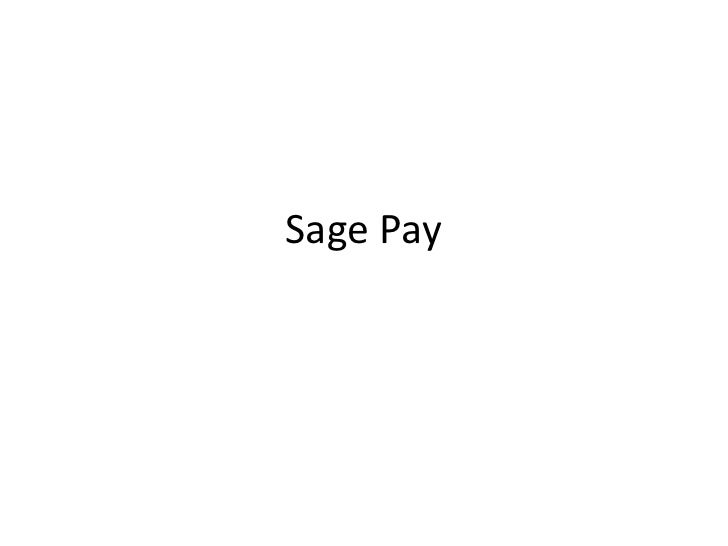The image features a plain white background with no discernible borders or perimeters. Positioned centrally within this vast expanse of white space, the text appears left-aligned. The text comprises two words: "SAGE" and "PAY," both written in average-sized black letters. The word "SAGE" is fully capitalized (S-A-G-E), while "PAY" starts with a capital 'P' (P-A-Y). There are no other elements or decorations in the image; just the simple, straightforward text "SAGE PAY" in black.